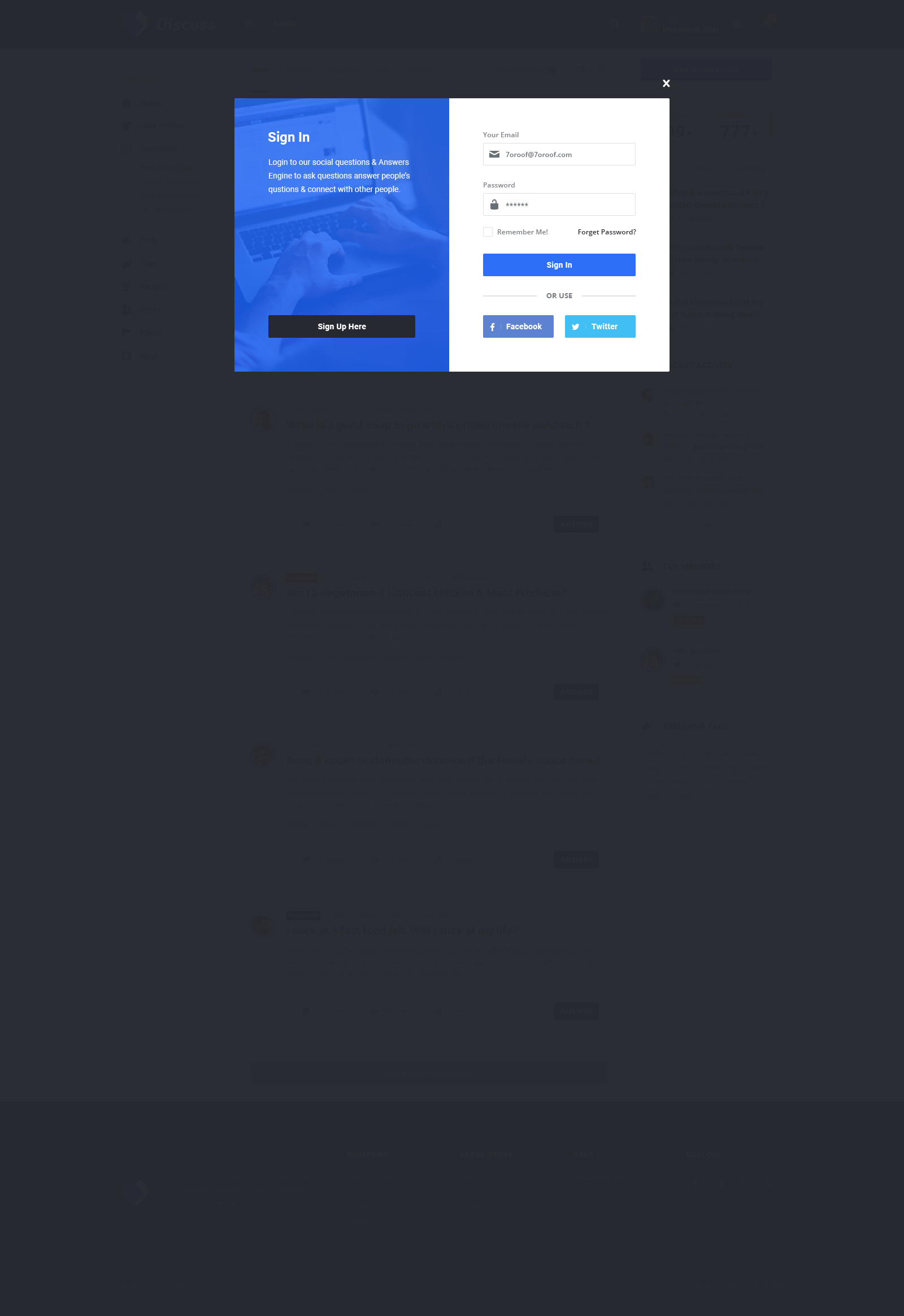The image features a dark, portrait-oriented background that is predominantly black. At the upper center of the image, there is a pop-up message with a white "X" in the top right corner, allowing users to close the message.

The pop-up is divided into two columns:
1. **Left Column:**
    - Title: "Sign In"
    - Description: "Log into our social questions and answers engine to ask questions, answer people's questions, and connect with other people."
    - The description phrase "to ask questions, answer people's questions, and connect with other people" is repeated for emphasis.
    - Background: A faint, light blue image of a person typing on a laptop.
    - Bottom: A black button labeled "Sign Up Here."

2. **Right Column:**
    - Background: Solid white.
    - Fields: 
        - Your Email (with a sample email: 7aroof@7aroof.com)
        - Password
        - Options: "Remember Me" and "Forgot Password"
    - Buttons: 
        - A light blue "Sign In"
        - Options to sign in using "Facebook" or "Twitter"
    
Additionally, the image hints at barely visible rows in the black background behind the pop-up, though they are not readable.

This visually contrasting image serves as a sign-in or sign-up interface for an online social platform aimed at fostering Q&A interactions.